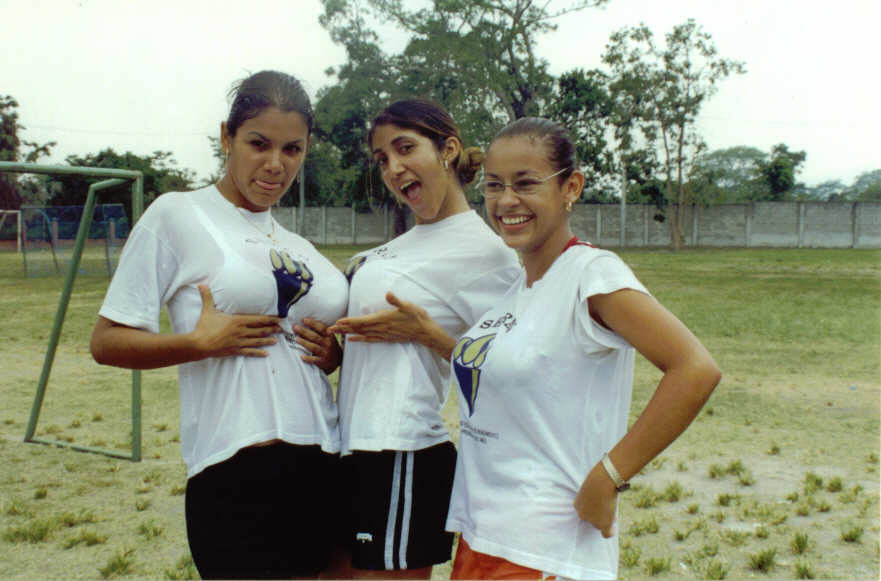In the image, three young women are standing in a grassy field with some short weeds, posing for the camera. They are all wearing white t-shirts and athletic shorts, with the one on the left sporting reddish-brown shorts and the other two in dark blue or black. Each t-shirt features what appears to be an image similar to an Olympic flame. 

The scene captures a playful moment as the women adopt various poses and facial expressions. The middle woman has her hands under her chest, pushing up her breasts, and her mouth open as if saying "Ah!" The woman on the left is sticking her tongue out slightly while looking mostly at the camera and similarly holding her chest. The woman on the right, wearing glasses, has her left hand on her hip and is smiling. 

In the background, there's playground equipment on the left, which might be a swing set, although the swings themselves are not visible. The field is trampled and weathered, bordered by a fence with trees beyond it. The sky is partly cloudy, appearing hazy and white with some patches of blue peeking through. The overall scene is one of youthful exuberance with a spontaneous, carefree vibe.